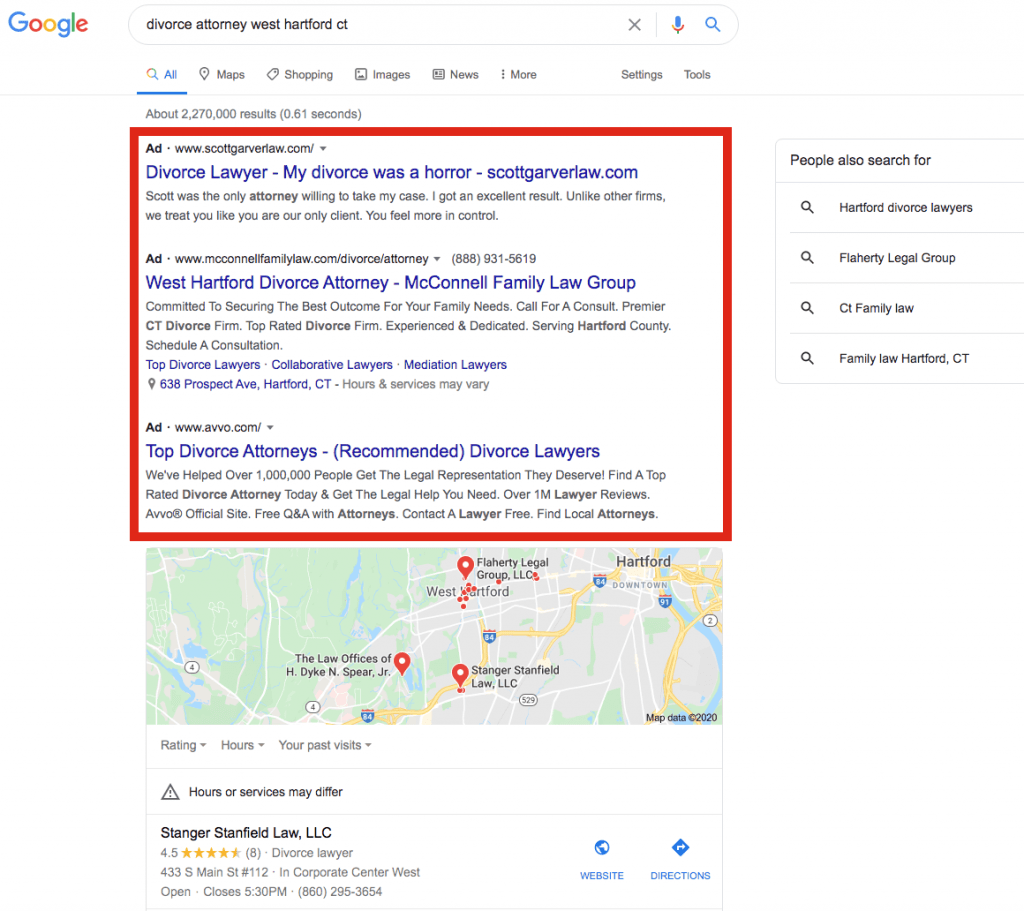A detailed and cleaned-up caption for the image could be:

"The image showcases a Google search results page for 'Divorce Attorney West Hartford CT,' highlighted with a white background. The search query itself is underlined in blue. The page displays various options including 'Maps,' 'Shopping,' 'Images,' 'News,' and 'More,' each accompanied by three vertical dots. A banner at the top indicates that approximately 2,270,000 results were found in 0.61 seconds. There is also a section titled 'People also search for,' featuring 'Hartford Divorce Lawyers' and three additional related topics. Below this, there is a red rectangle highlighting three specific websites: 'Divorce Lawyer,' 'My Divorce Was A Hard.com,' and 'Scott Garver Law.com,' followed by 'West Hartford Divorce Attorney, McConnell Family Law Group.' Additionally, in blue text, there are sections for 'Divorce Lawyers,' 'Collaborative Lawyers,' and 'Mediation Lawyers,' along with a mention of 'Top Divorce Attorneys (Recommended).' A picture of a map displaying three location icons is visible, with information about rating, hours, and past visits. A triangle icon with an exclamation mark warns that 'Hours or services may differ.'"